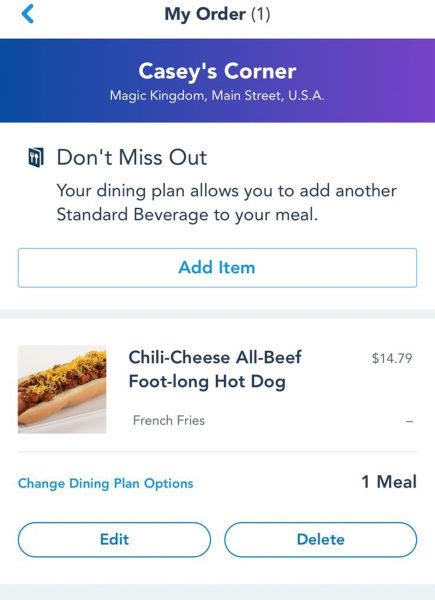A cropped screenshot from the **My Disney Experience** app’s mobile order section for Disney World, displaying details for an order at **Casey's Corner** in **Magic Kingdom** on **Main Street USA**. 

At the top, "My Order (1)" is prominently shown in large blue font, with a left-pointing arrow on the far left. Below is a large purple banner reading "Casey's Corner Magic Kingdom Main Street USA" in centered text. 

Further down, a blue header declares "Don't Miss Out," followed by a message stating, "Your dining plan allows you to add another standard beverage to your meal." A white bar below this provides an "Add Item" option. 

Displayed beneath is the first menu item: a thumbnail image of a footlong hot dog on the left. To the right, the item is described as a "Chili Cheese All Beef Footlong Hot Dog," with "French Fries" noted beneath in small grey text. The price of $14.79 is listed to the right of the item name. At the bottom left, a light blue text option reads "Change Dining Plan Options," while the bottom right corner shows "1 Meal" in large grey font.